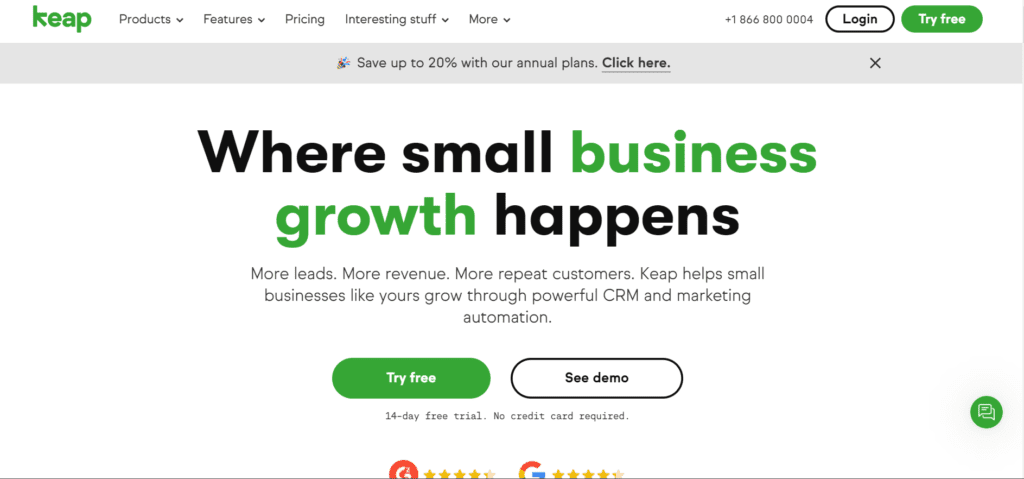The website homepage prominently features "KEAP" in green text, with a grey navigation bar that includes options for "Products," "Features," "Pricing," "Interesting Stuff," and "More." The "Pricing" section appears to be selected, indicated by a down arrow beside it. The webpage also displays a contact number, "1-866-800-0004," and offers options to "Login" and "Try Free." The "Login" button is placed on a white rectangle, while the "Try Free" button is on a green rectangle.

The headline reads, "Where Small Business Growth Happens," followed by subheadings emphasizing the benefits such as "More Leads, More Revenue, More Repeat Customers." The description highlights that KEAP helps small businesses grow through powerful CRM and marketing automation tools.

Additionally, there is a call-to-action with two buttons: "Try Free" on a green rectangle and "See Demo" on a white rectangle. The page offers a "14-day free trial, no credit card required." At the very top of the page, there is an offer stating "Save up to 20% with our Annual Plans" with an underlined "Click Here" hyperlink, indicating it is clickable. An 'X' for closing the offer or pop-up is located off to the right.